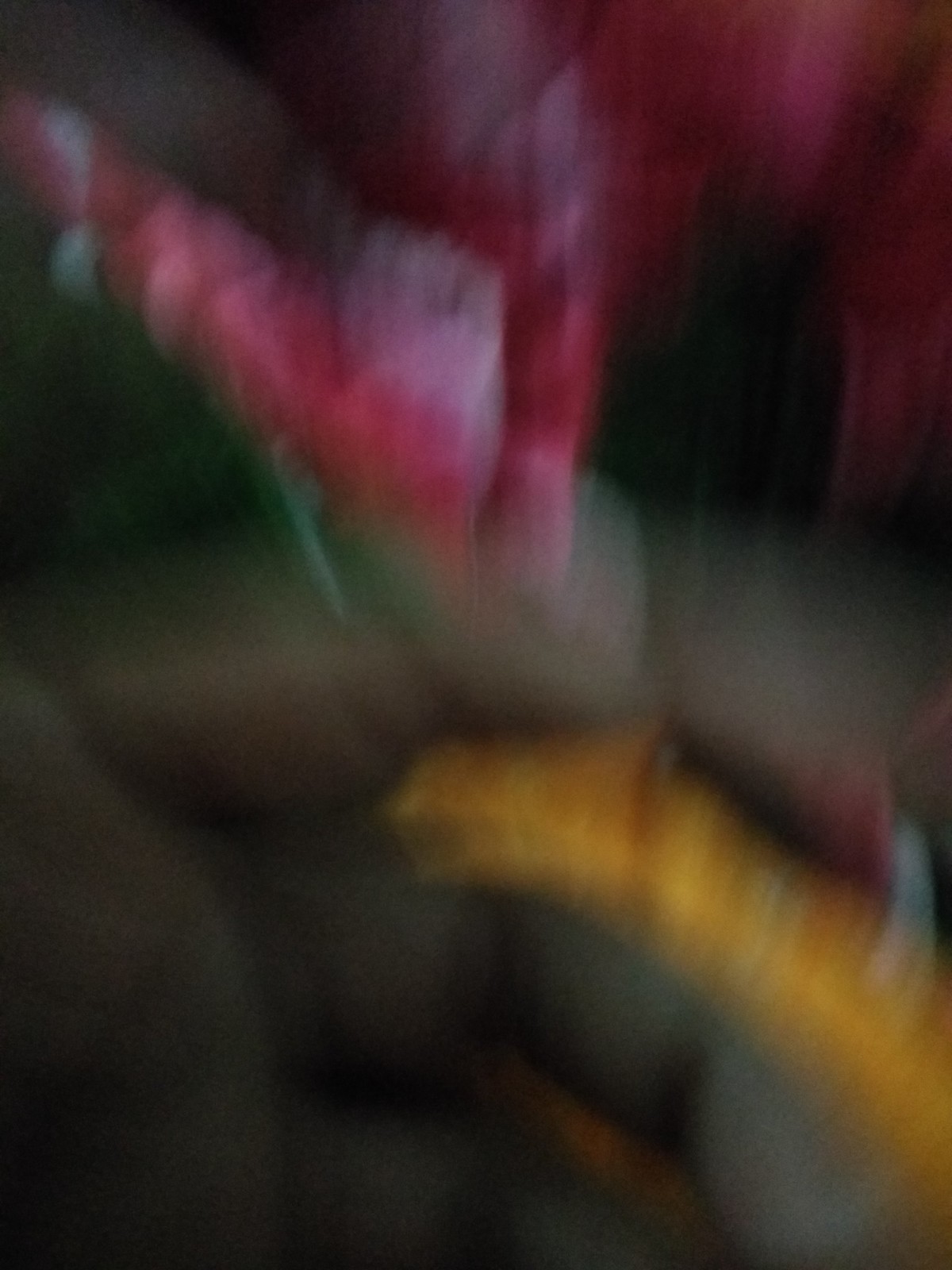This image is extremely blurry and out of focus, rendering details difficult to discern clearly. Dominating the bottom half of the photo is the palm of a person's hand, with fingers bent and extending towards the right. The top portion of the palm nestles under the curved fingers. A bright yellow object, possibly a root or similar-looking item, is visible between the index and middle fingers. Above this, a pink element descends from the top left, makes a V shape, and then ascends again before trailing down the right side. The image also reveals the knuckles at the base of the fingers.